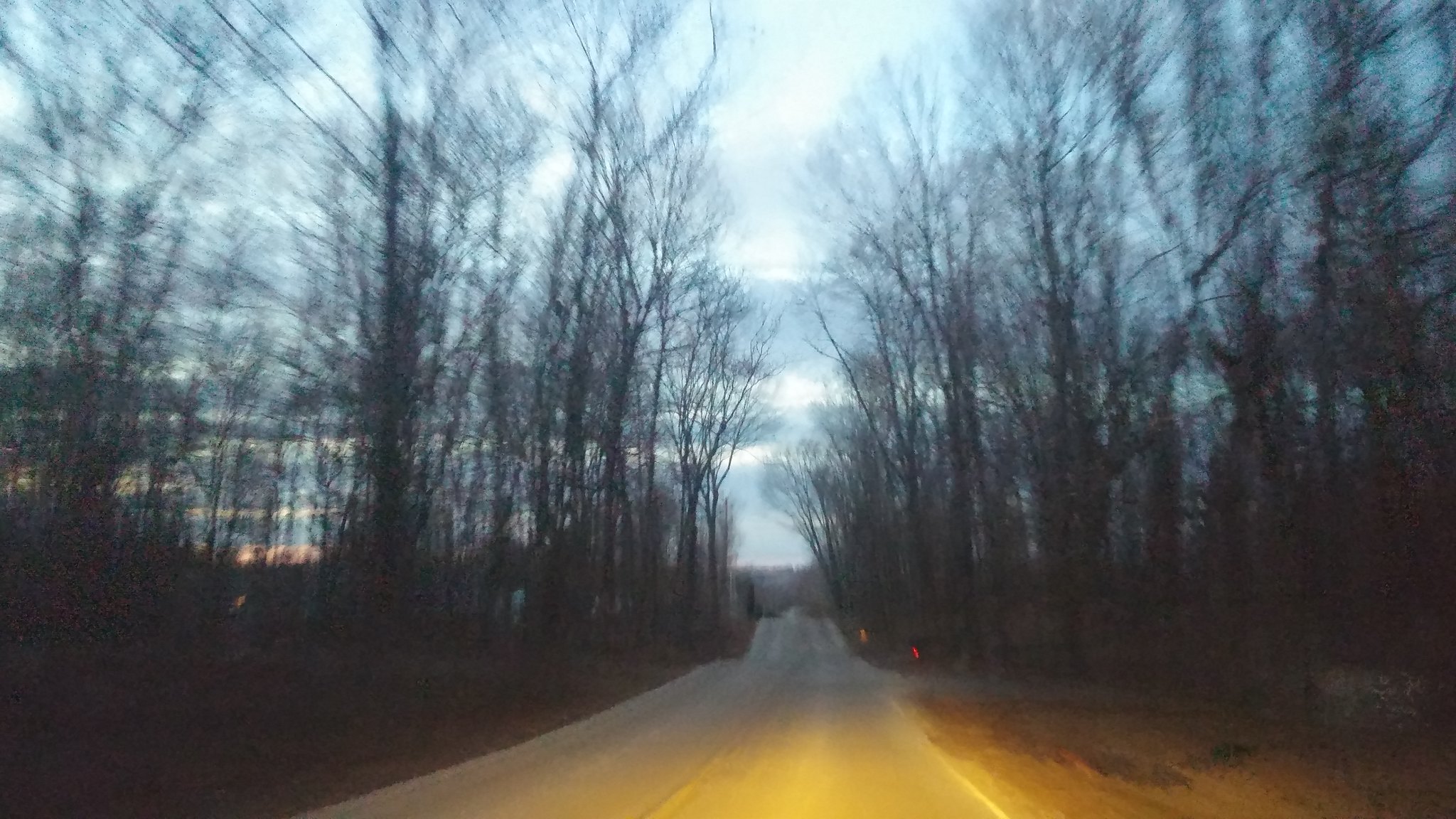A vibrant image captures a serene two-lane road slicing through a dense forest, embodying the photographic concept of a vanishing point. The forest stretches from the lower left, through the center, to the lower right-hand corners of the frame, forming a natural tunnel of greenery. The road is distinctly marked by a double yellow line, signifying two-way traffic, with our lane on the right and opposing traffic on the left. Crisp white lines border each side of the road, hinting at narrow shoulders or walking lanes meant to keep vehicles centered. Reflective markers punctuate the right-hand shoulder, enhancing visibility. The image, possibly taken from a moving car, showcases a stretch of road bathed in gentle light, leading the eye toward the distant horizon where the road meets the sky.